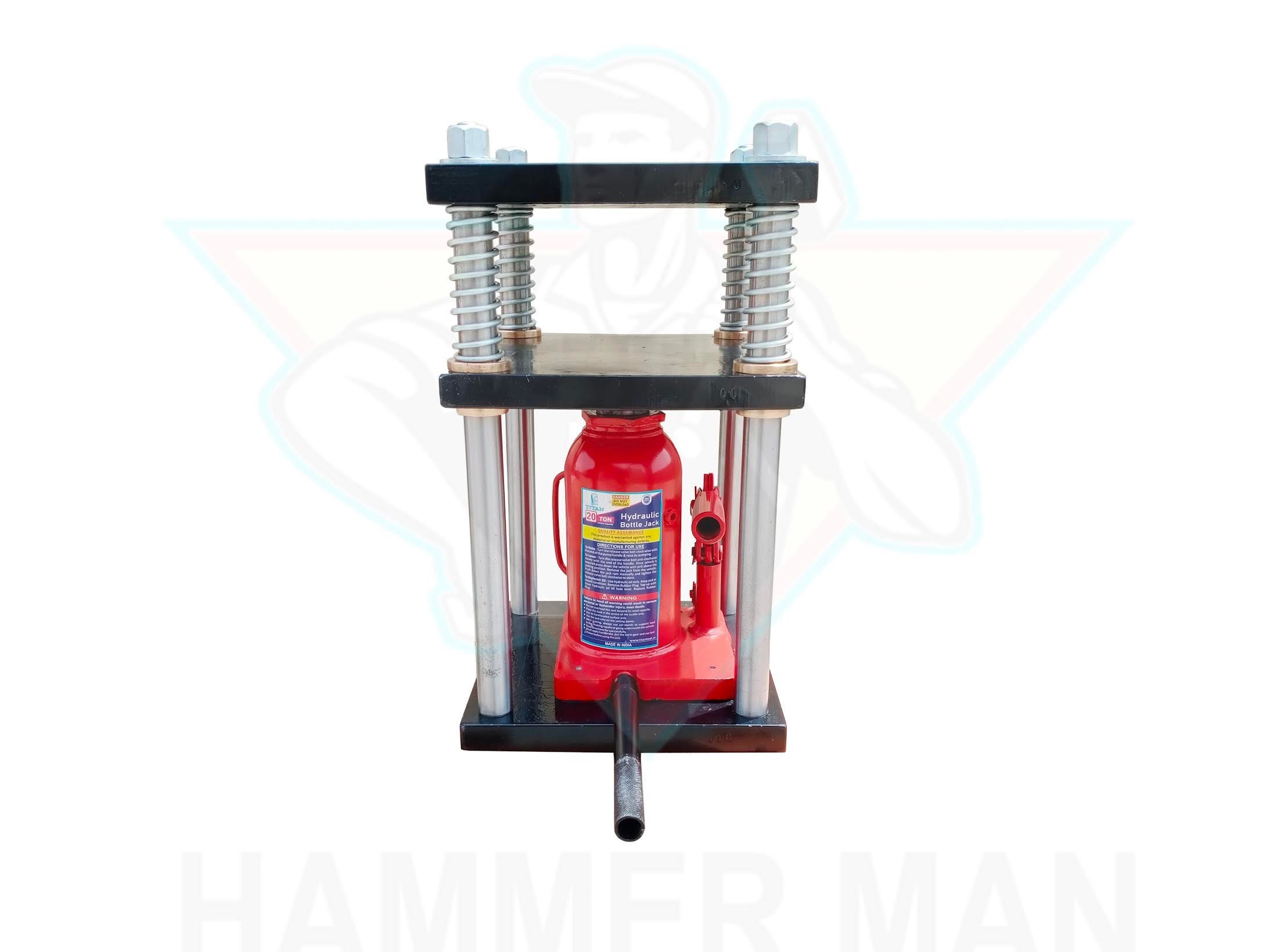This image features a two-tiered metal shelf supported by four polished silver columns with bolts and springs at the top. The spacing of the shelves creates three layers. The shelves themselves appear to be sturdy, painted in black, possibly metal or stone, and giving an impression of heaviness. Situated prominently on the bottom tier is a red cylindrical device identified as a hydraulic bottle jack or a gas dispenser, characterized by a black handle or tube protruding from it. It also includes a blue label without clear instructions and appears to have an incomplete attachment, suggesting it might be a housing unit for the tool. The background features a watermark with the text "Hammer Man" and a logo depicting a man wearing a baseball cap, raising a hammer, encapsulated within a tri-colored triangle. The entire background of the image is white, providing a clear contrast to the foreground elements.